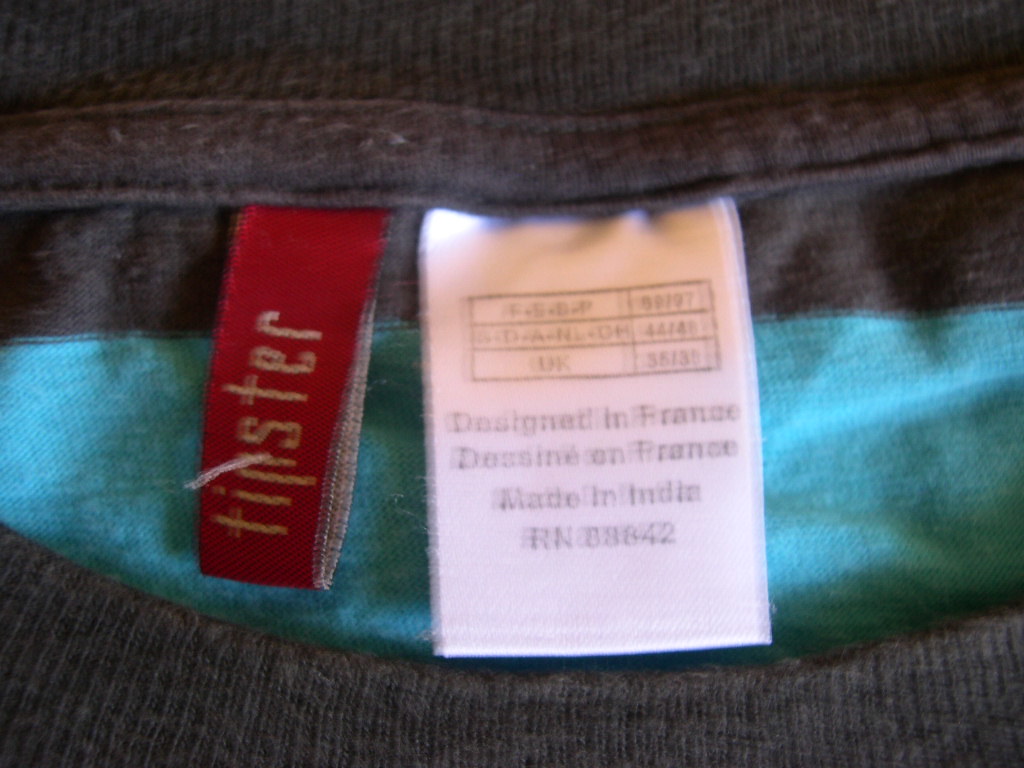The image showcases an extreme close-up of a clothing tag attached to a sweater-like garment. In the lower section of the image, the texture of the fabric is prominently visible, characterized by a rich black and dark gray knit pattern. A notable feature in the center of the image is a blue oval shape that casts a subtle shadow on the fabric. To the left, there is a vertical red tag with the word "tinster" written in a yellowish color. On the right side, a white, square-shaped tag displays a size chart with the inscriptions "Designed in France," "Made in India," and "RN 03642." The upper section continues the display of the dense, cozy knit texture that extends throughout the image.